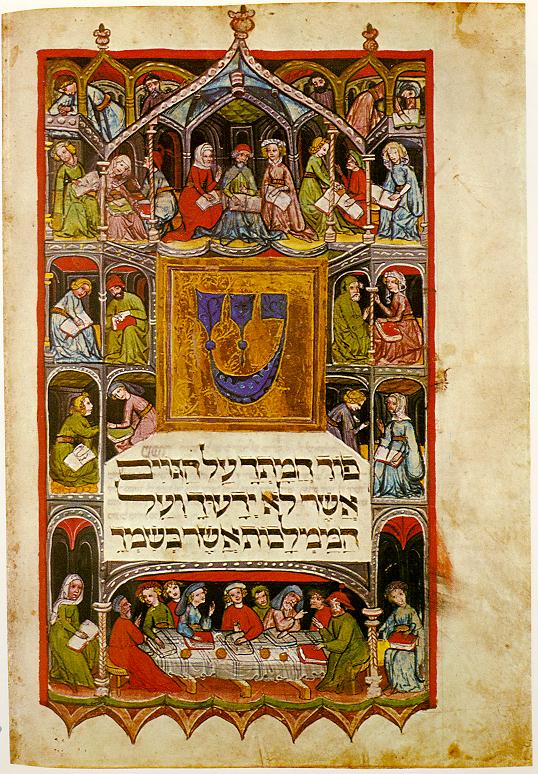The image depicts an aged piece of beige parchment, yellowed with time, that appears laden with historical and religious significance. Centered on the parchment, slightly toward the bottom, is an elaborate, hand-drawn illustration adorned with vibrant, predominantly red and green hues. It portrays a multi-layered architectural structure teeming with various figures engaged in discussions, many of whom are holding pillows. Scattered throughout the parchment, there are handwritten Hebrew characters, enhancing the artifact's Middle Eastern or Judaic aura.

Prominently at the bottom of the illustration, a group of individuals, reminiscent of the Last Supper, are seated around a long, rectangular table, deeply engrossed in conversation. The attire of the figures—long, floor-length robes—further underscores the religious context of the scene, evoking historic religious traditions. The parchment's wear, including noticeable staining and yellowing, suggests it has been passed through various hands over the years, adding a palpable sense of antiquity and reverence.